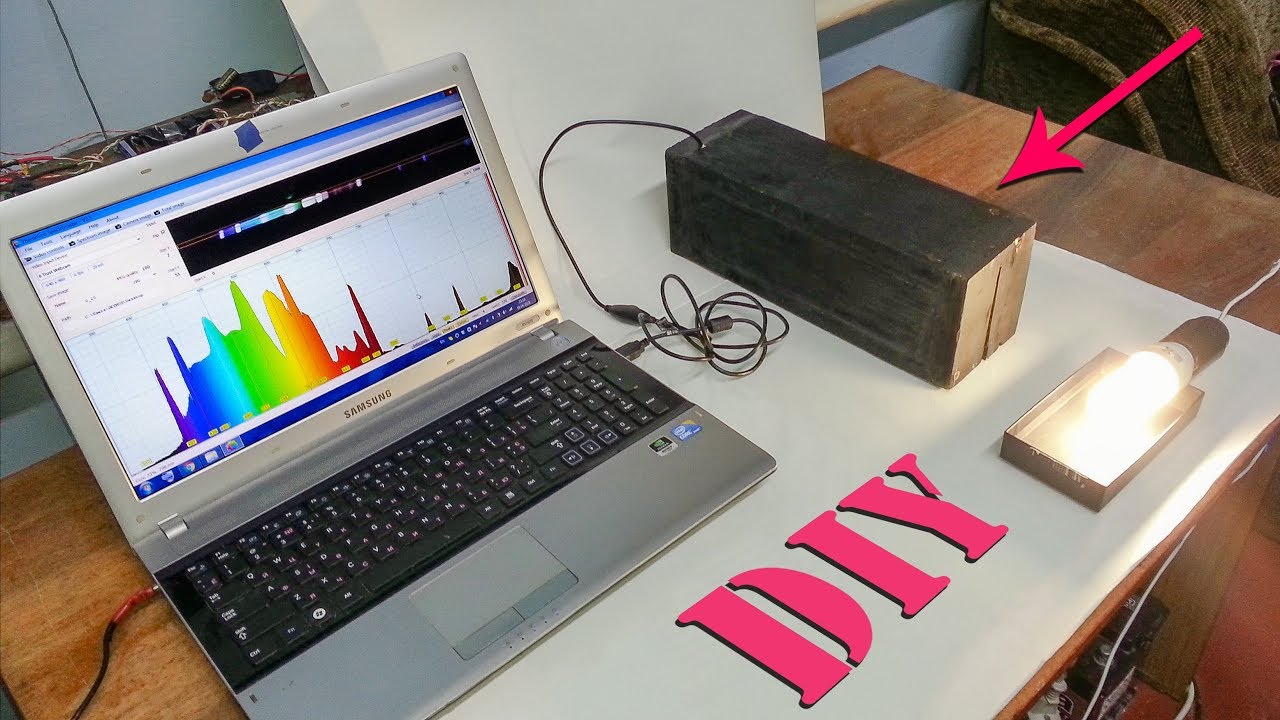This photograph showcases a scientific project spread across a natural brown, wooden desk. Dominating the left side of the table is a silver Samsung laptop with a black built-in keyboard featuring white lettering on the keys. A small piece of blue tape covers the laptop's camera. The laptop screen displays a rainbow-colored graph, possibly analyzing wavelengths or light frequencies. Below the laptop, there's a white sheet adorned with the pink letters "DIY." Connected to the laptop via a USB cable is a black-painted wooden box. To the right of this setup, a lit bright white light bulb is connected by a white wire and positioned on a square-shaped white surface. Additionally, in the top right corner of the image, a pink arrow points towards the black box, emphasizing its significance in the project.